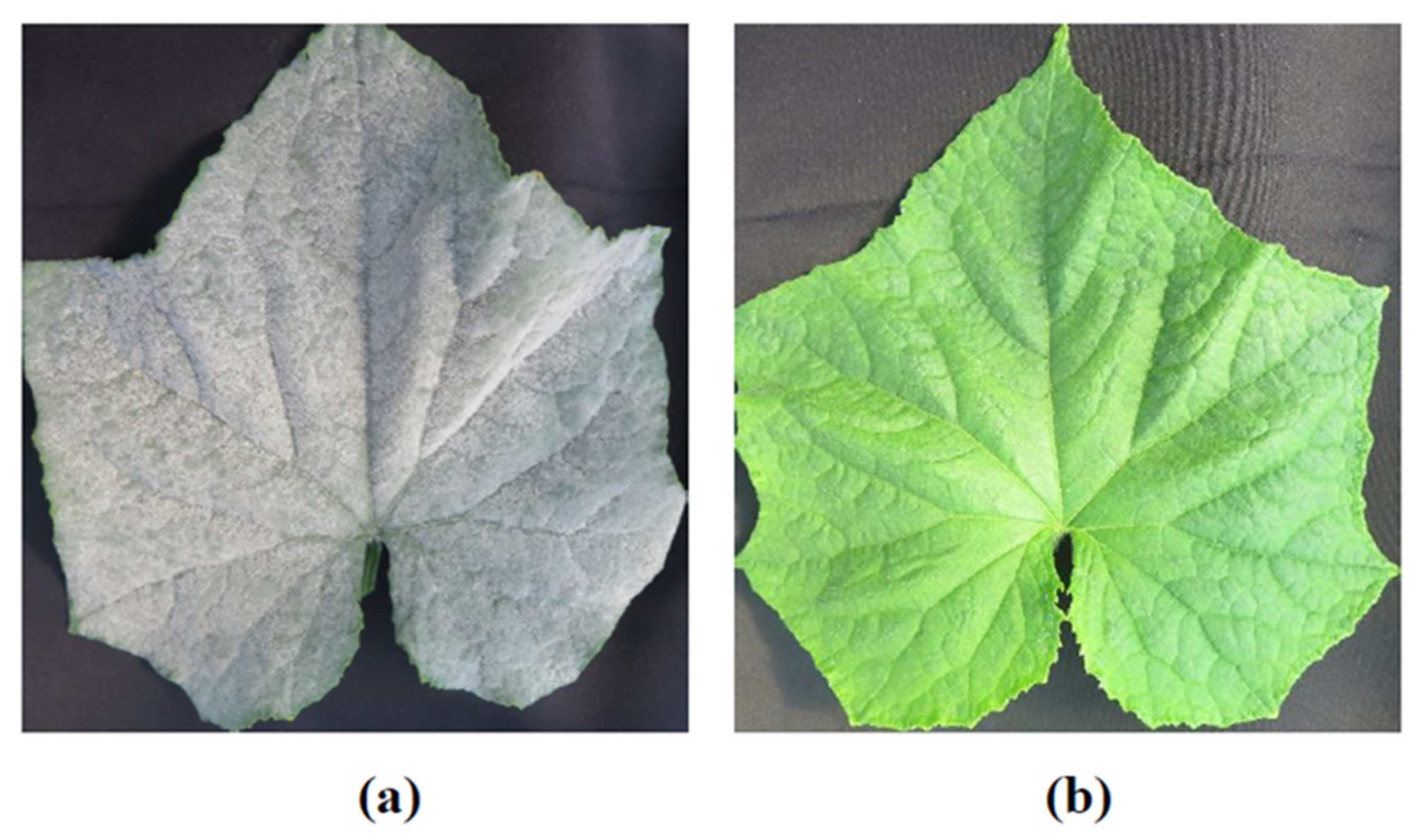The image consists of two side-by-side photographs of similar-shaped leaves, labeled A and B respectively. The leaf in photo A, on the left, is depicted in black and white, showing a range of gray tones with visible veins, and seems to be mottled with patches of lighter and darker shades, potentially indicating disease. Contrarily, the leaf in photo B, on the right, is shown in color and appears healthy, displaying a vibrant, muted green hue with a slight tinge of yellow, reflecting light to highlight its glossy surface. Both leaves feature a distinctive shape with five radiating, pointed spokes extending from a rounded base to a noticeable tip. The background for both images is simple and dark, providing a stark contrast that emphasizes the details and textures of the leaves. The lighting is direct and head-on, clearly illuminating the leaves' vein structures.